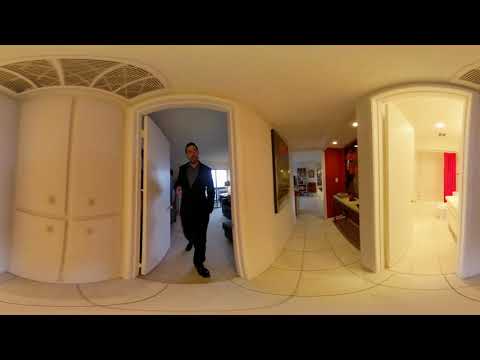The panoramic image, bordered thickly in black at the top and bottom, showcases a man in profile as he steps through an open doorway situated on the left side of the frame. He is dressed in a black suit jacket, dark pants, and dark shoes, with a blue shirt under the jacket and short black hair. His right foot is forward, suggesting his imminent exit from a bright room illuminated by daylight streaming through a window behind him. 

The setting is a hallway branching into various directions, characterized by cream or white decor and a floor patterned with darker linear gradients forming square shapes. On the right side of the hallway, a door swings inward to reveal a bathroom with a red shower curtain pulled to one side, exposing the shower, toilet, and the edge of a sink. The image's warped perspective, indicative of a 360-degree video frame laid flat, gives the scene a curved, distorted appearance, particularly noticeable in the rounded lines between the white floor tiles. To the right of the central hallway, another door opens into a room with red curtains. The left-hand side of the frame reveals sections of furniture and wall decorations, blending into the overall warped and elegantly styled environment.